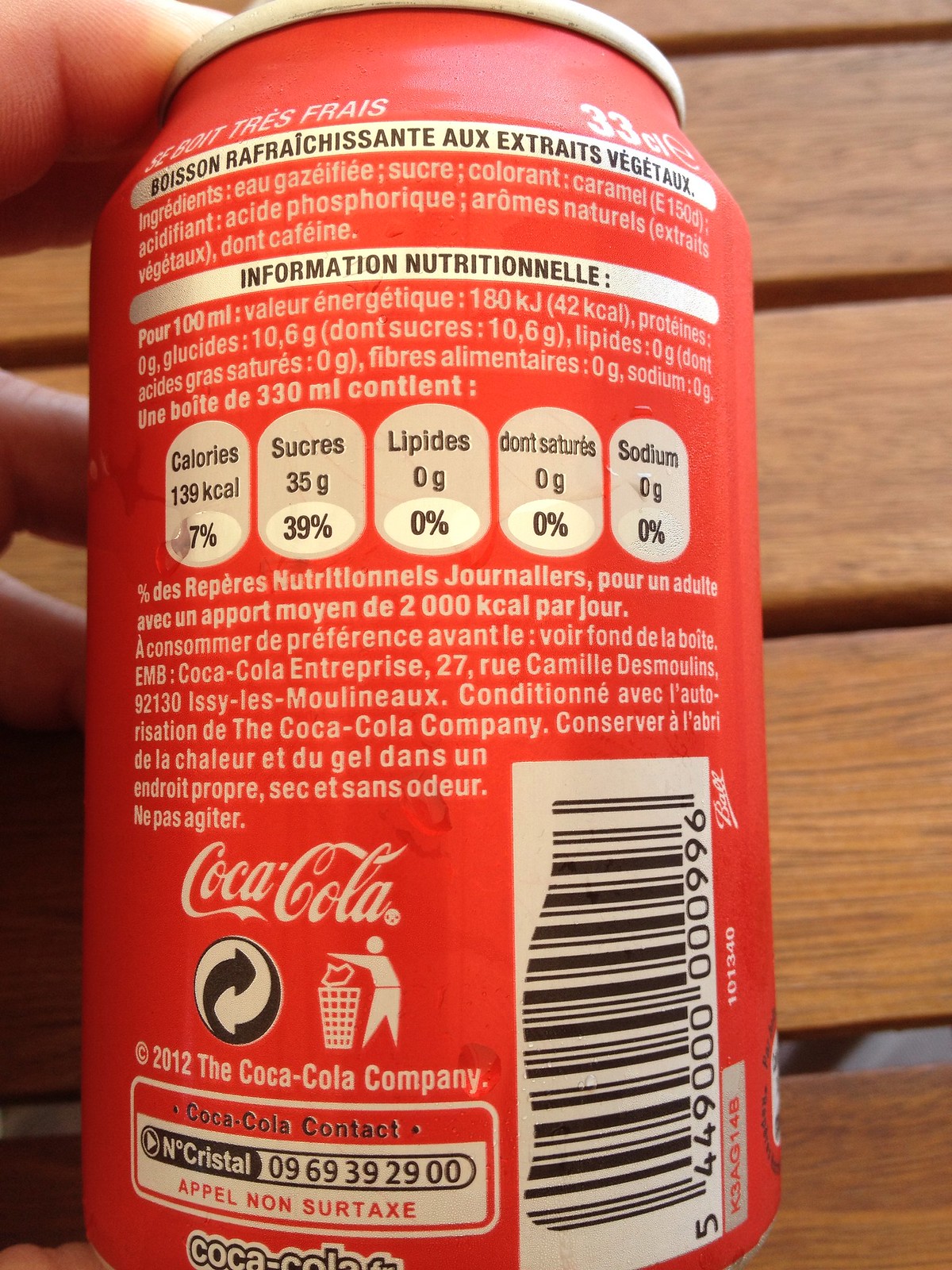In this image, we see the back of a cylindrical can with a person's fingers touching it from the top left corner. The can's side is prominently colored red. The label on the can features text in a foreign language, rendered in black and white. Across the top, the text reads "SE BOIT TRÈS FRAIS," which suggests that the beverage is best served cold. On the top right, it is marked with "33 CL E," indicating the can's volume. Below, the label reads "BOISSON RAFRAÎCHISSANTE," which translates to "refreshing drink."